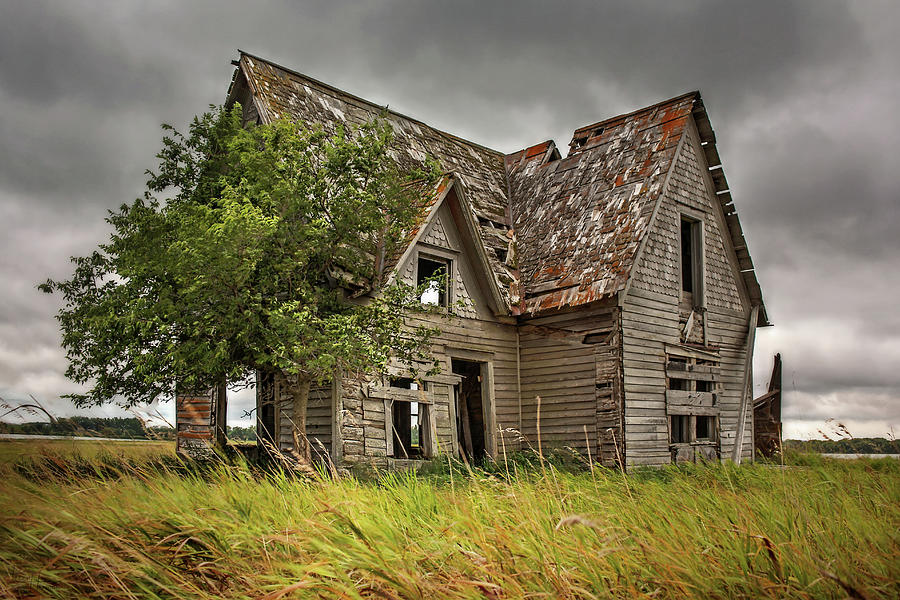This striking image captures either a photograph or a meticulously detailed painting of an old, abandoned farmhouse situated in the rural Midwest United States. The house, made of wood, stands as a two-story structure, though it appears rickety and dilapidated with numerous boards and shingles missing from its slanted roof. The chimney is notably absent, leaving a gaping hole where it once stood. Busted windows and doors, some boarded up, offer a haunting glimpse through to the other side of the house. Dominating the foreground is a field of tall green grass, with a large, imposing tree on the left side adding to the scene's rustic charm. Dark gray skies with menacing clouds hover above, casting an eerie ambiance over the landscape. In the distance, occasional trees dot the horizon, emphasizing the isolation and forlorn state of this once charming farmhouse.